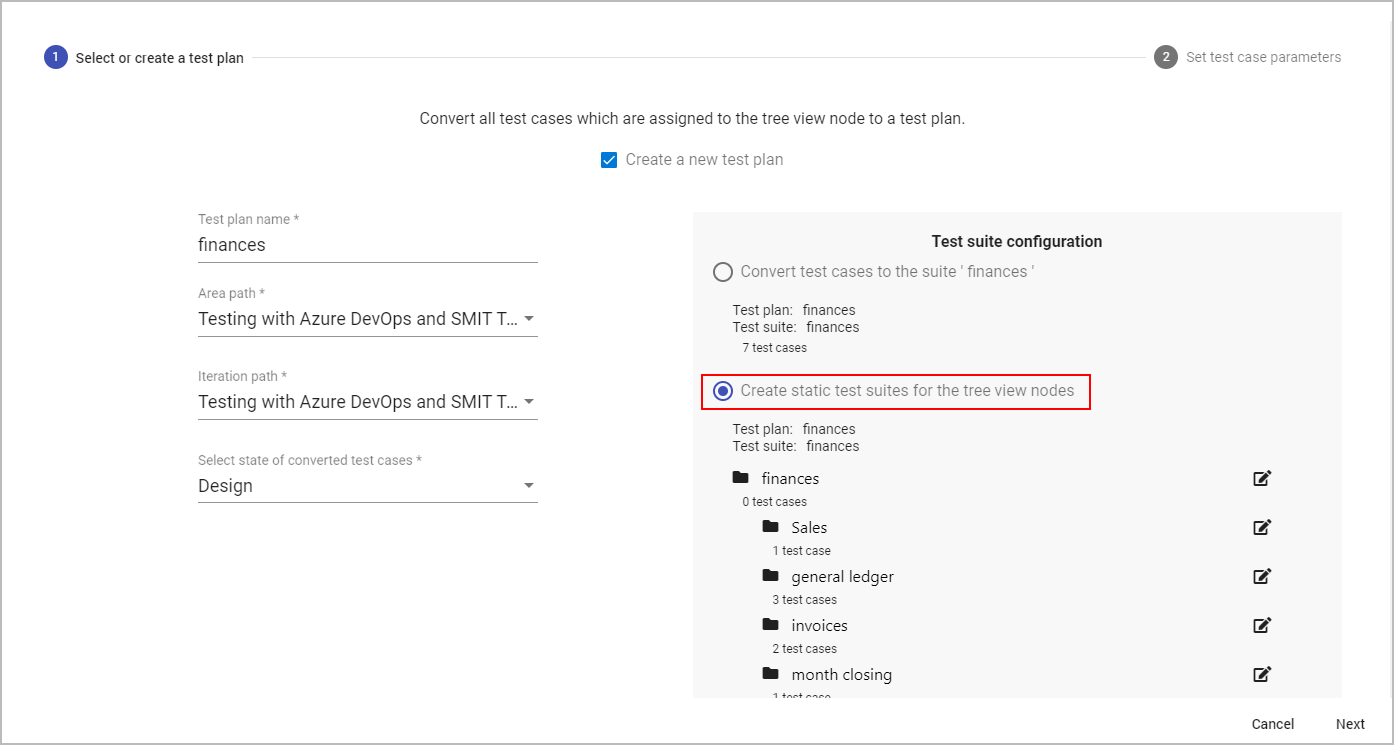The image appears to be a screenshot of a computer interface, likely displaying a guide or a tool for managing test plans and cases. The background is predominantly white with sections of black text and various interface elements.

In the upper-left corner, a blue circle with the number "1" is visible next to the text: "Select or create a test plan." Extending from this point, a horizontal line goes across to the right side of the screen, leading to a gray circle with the number "2." Next to this circle, the text reads "Set test case parameters."

At the center of the screen, there is a prominent title in bold, stating: "Convert all test cases which are assigned to the tree view node to a test plan." Beneath the title, a blue box with a checkmark is labeled "Create a new test plan."

On the left side, the interface includes several fields:
- "Test Plan Name" filled with "Finances"
- "Area Path" filled with "Testing with Azure"
- Additional unspecified entries

On the right side, a gray box titled "Test Suite Configuration" is present. Inside this box, there is a clickable circle option with unclicked text reading "Convert test cases to the suite finances." Below this, another clickable option features a blue circle with a red outline around the text: "Create static test suites for the tree view nodes." Additional text and options are listed underneath.

The overall layout of the screenshot indicates a structured process for creating and configuring test plans within a software development or testing tool.